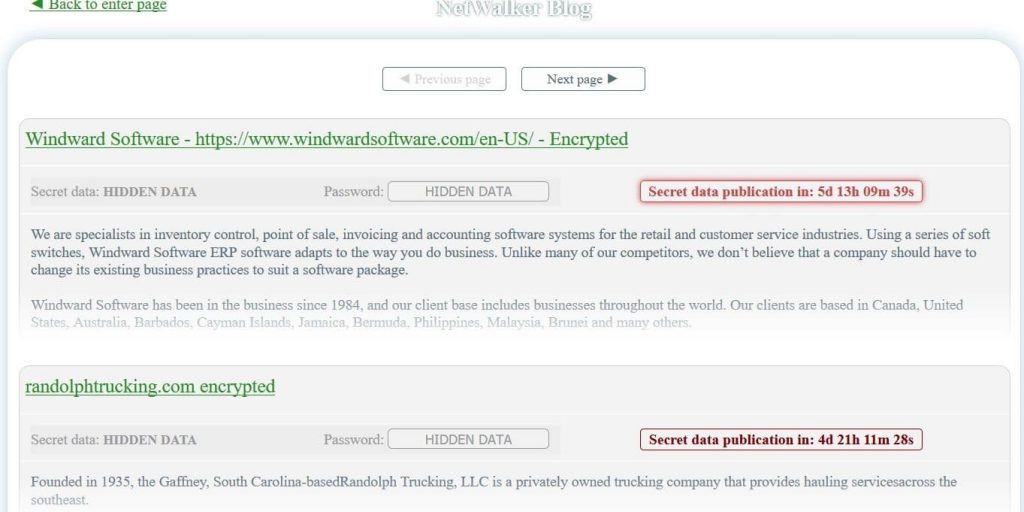In the top left corner, in green text, it says "Back to Enter Page" accompanied by a small arrow pointing left. To the right, in very light gray text, the words "NetWalker Blog" are displayed. Directly beneath this, there is a rectangle with faint text saying "Previous Page," and next to it, in a bolder color, is another rectangle with the text "Next Page" and an arrow pointing right.

Below this, a green and underlined hyperlink reads "Wind Software - www.windwardsoftware.com - EN - US - ENCRYPTED". Moving down and to the right, inside a small red rectangle, it says "Secret Data Publication in 5d 13h 09m 39s".

Continuing downward on the left side, in green underlined text, it states "RandolphTrucking.com - ENCRYPTED". To the right of this, within another rectangle, it notes "Secret Data Publication in 4d 21h 11m 28s".